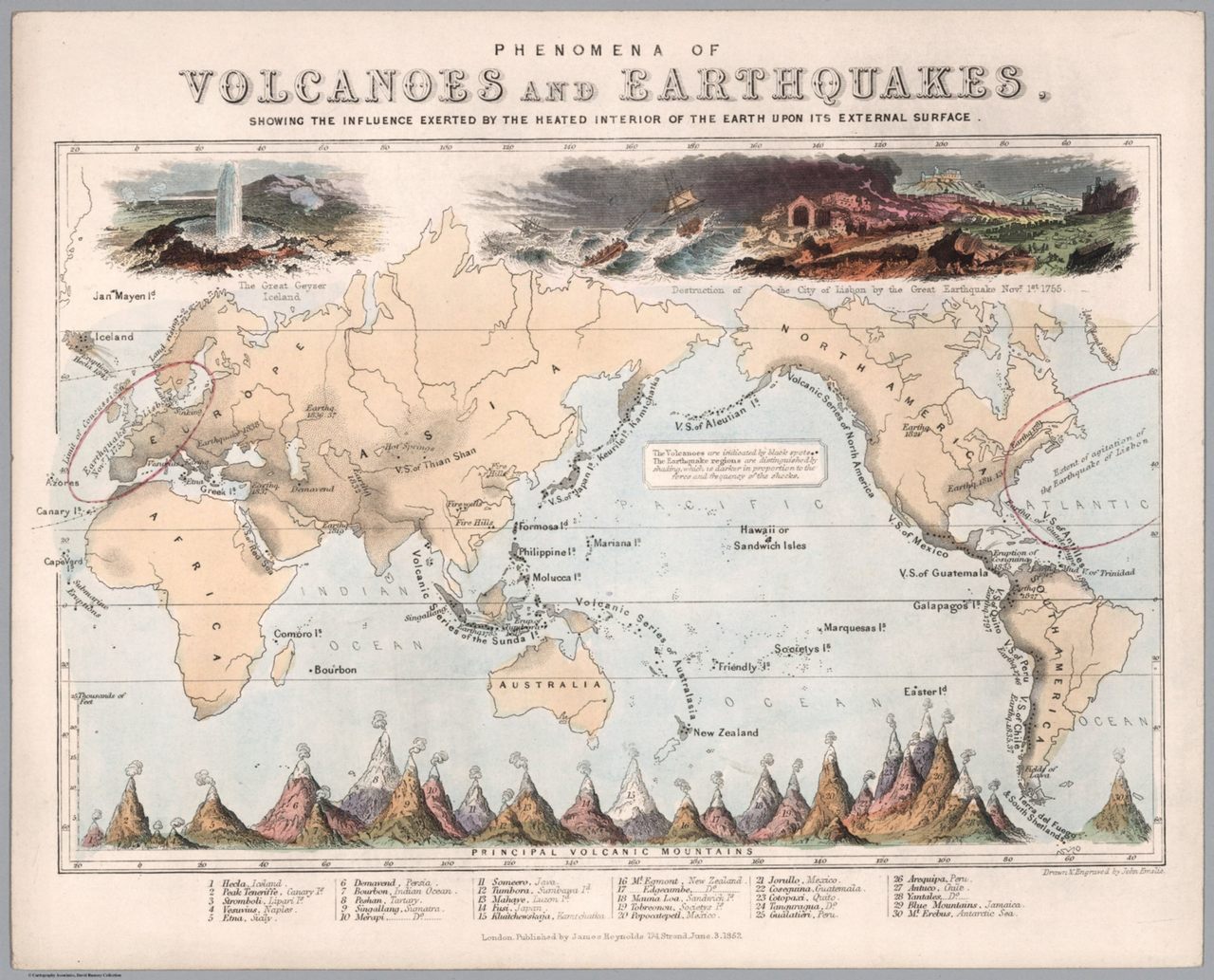This image presents an intricate and historical art piece combined with a map, rendered on a light cream-colored paper. At the top, in black text, it reads "Phenomena of," followed by the prominent and artistic title "Volcanoes and Earthquakes" in much larger font. The full heading reads: "Phenomena of Volcanoes and Earthquakes, Showing the Influence Exerted by the Heated Interior of the Earth upon Its External Surface."

The main feature of the image is a detailed world map, with all continents labeled and surrounded by oceans depicted in a light blue color. Above this central map, but below the heading, there are artistic representations of natural phenomena, possibly drawn or painted in pencil or paint. These illustrations include erupting volcanoes and turbulent seas with boats, capturing the dramatic effects of natural forces.

Below the map, the image portrays vibrant shapes resembling mountains, rendered in shades of purples, pinks, oranges, and greens. There is also a legend provided at the bottom, which appears to categorize various types of mountain peaks and lists principal volcanic mountains numbered from 1 to 30, although the text in this section is too small to be read clearly from the image.